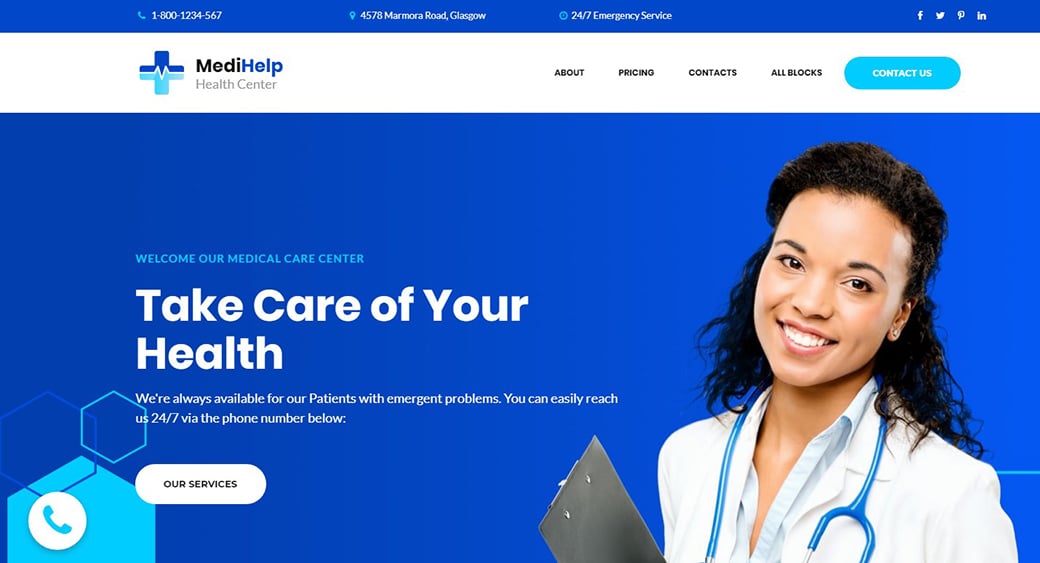A detailed screenshot of the Medihelp Health Centre website highlights its professional and accessible design. The website's title, "Medihelp Health Centre," is prominently displayed near the top left of the page. The colour scheme is primarily royal blue, exuding a sense of trust and professionalism.

At the top, a blue information bar features a telephone icon alongside the contact number and the centre's address: 4578 Manorka Road, Glasgow. An icon indicating 24/7 emergency service is also present. To the right of this bar, the social media icons for Facebook, Twitter, an unidentified platform, and LinkedIn are shown.

Beneath the information bar is a white navigation bar, featuring the title "Medihelp Health Centre" and the centre's logo—a blue cross with the top part in dark blue, the bottom part in light blue, intersected by a diagonal line resembling a heart rate monitor.

The navigation menu includes links to About, Pricing, and Contacts, all in white boxes, accompanied by a light blue "Contact Us" button. The main section of the page is dominated by a large background photo. On the right side of this photo, a young black woman, dressed as a doctor in a white coat with a stethoscope around her neck, smiles warmly at the camera, making her appear approachable and trustworthy.

The page's main title, "Take Care of Your Health," is prominently centered and accompanied by the subtitle, "Welcome to our medical care centre," in smaller text. Below, the phrase "We're always available for our patients with emergent problems. You can easily reach us 24/7 via the phone number below" assures visitors of the centre's constant availability. A white button labeled "Our Services" and a phone logo at the bottom left complete the page's call-to-action elements.

Overall, the screenshot presents a clear and inviting advert or homepage for the Medihelp Health Centre, emphasizing emergency accessibility, professional care, and easy contact options.